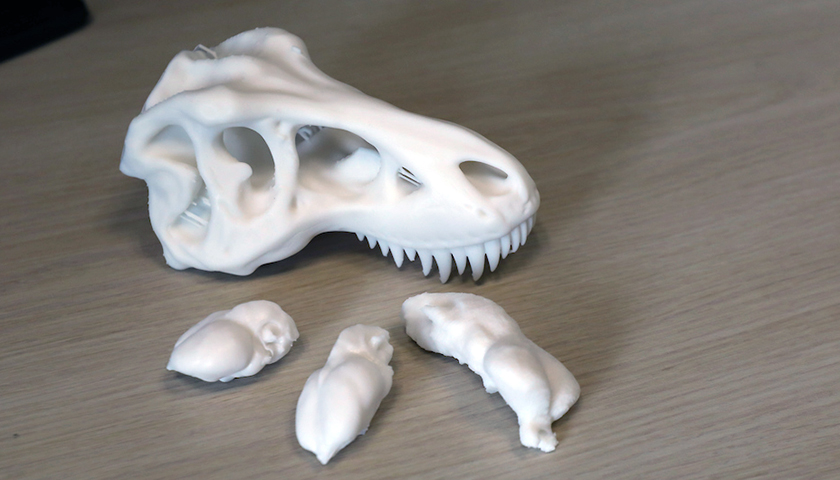The image depicts what appears to be a remarkably pristine and highly detailed dinosaur skull, specifically the top half with the upper jaw and sharp, white teeth perfectly preserved. The skull, exhibiting eye sockets, a nose channel, and three ridges on top, likely represents an archaeologically significant find. However, its snow-white color and the flawless condition raise skepticism about its authenticity, suggesting it may be handmade or 3D printed rather than an original bone structure. Inside the skull, remnants of plastic or paper hint at it being a constructed model. Positioned on a beige/light brown wooden table, the scene is lightly shadowed, adding to the curiosity. Accompanying the skull are three enigmatic white objects, identical in material and color, possibly resembling broken jaw fragments or internal organs, placed near the skull's teeth area. Their exact purpose remains unclear, contributing to the overall mysterious and somewhat artificial feel of the setting.